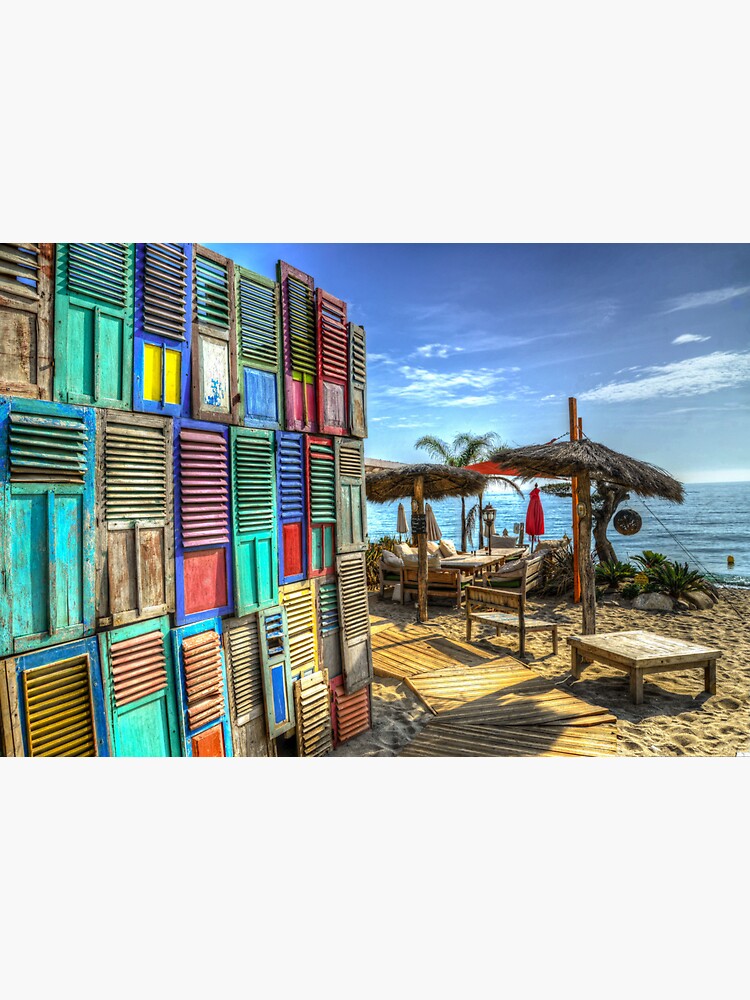A vibrant beach scene unfolds under a sunny, blue sky adorned with wispy white and a few puffy clouds. The tranquil blue water meets a well-trodden sandy shoreline, scattered with various pieces of wooden furniture including stools, benches, and tables. A distinctive feature is the wall on the left lined with doors, some with bright shutters, painted in a kaleidoscope of colors - turquoise, yellow, blue, pink, green, and purple. This colorful wall, perhaps an artistic installment or a row of locker doors, delineates the beach from the area beyond. Small wooden poles topped with dark brown and gray straw mushroom caps dot the sandy area, adding to the tropical ambiance. Visible are several large umbrellas, both open and folded, and a red umbrella near the water. There’s also a buoy floating peacefully in the distance. A boardwalk made of wooden pallets curves through the scene, guiding visitors towards the heart of this idyllic beach setting.